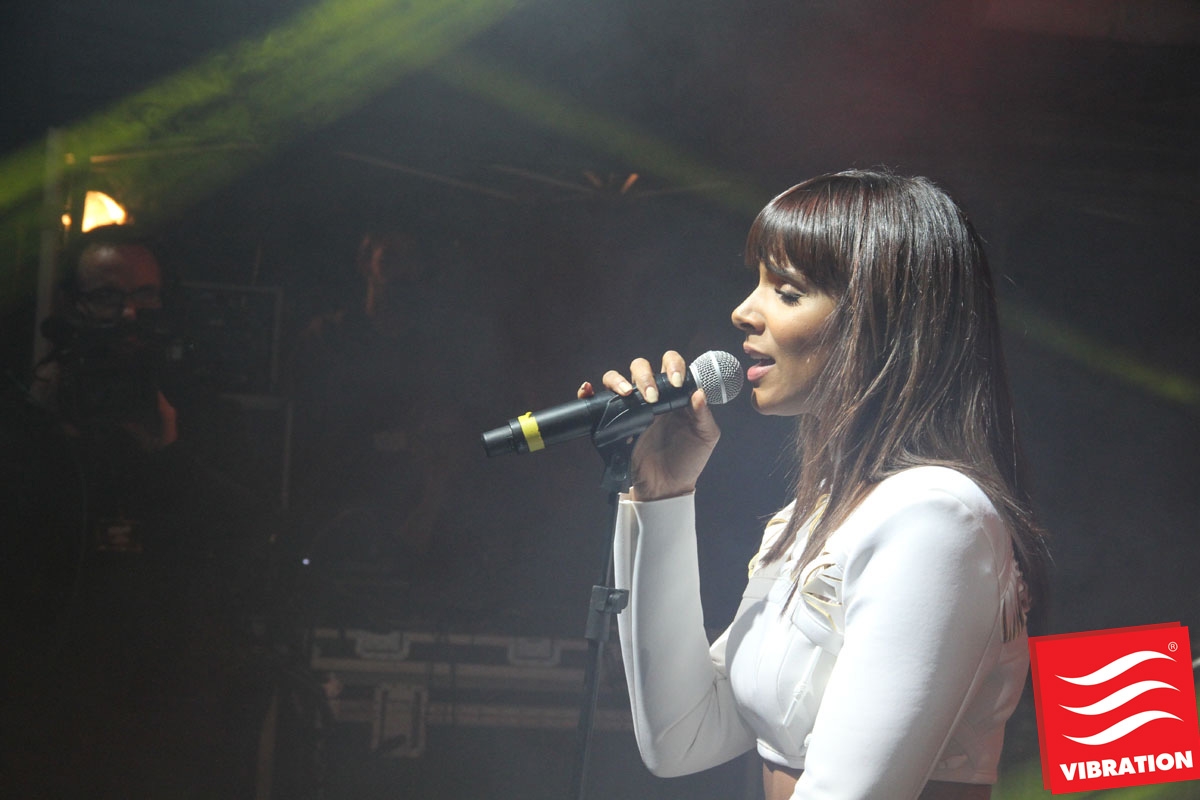This image captures a medium dark-skinned singer on stage, facing left, her left shoulder nearest to the camera. She has long, straight brown hair that reaches just past her shoulders with short bangs, and she is dressed in a white, long-sleeve crop top that reveals a hint of her midriff. The singer's eyes are closed as she passionately holds a microphone at her lips with her right hand, elbow bent. 

The stage around her is dimly lit, adding to the focused ambiance. To the right of the singer, there’s a red, slightly tilted square with three white wave icons and the word "vibration" underneath, likely a logo or watermark. In the background, shadowy figures hint at the presence of other people, possibly band members, stage technicians, or perhaps an audience. Among them, to the left, there's a cameraman with black, slightly receding hair and glasses visible above the camera he is using, further suggesting this might be a recording rather than a live performance. Positioned alongside him is another individual, also on stage, amidst musical equipment and subtle lighting effects that may include faint smoke or fog. The setting overall blends both a performance and a possibly intimate recording environment.